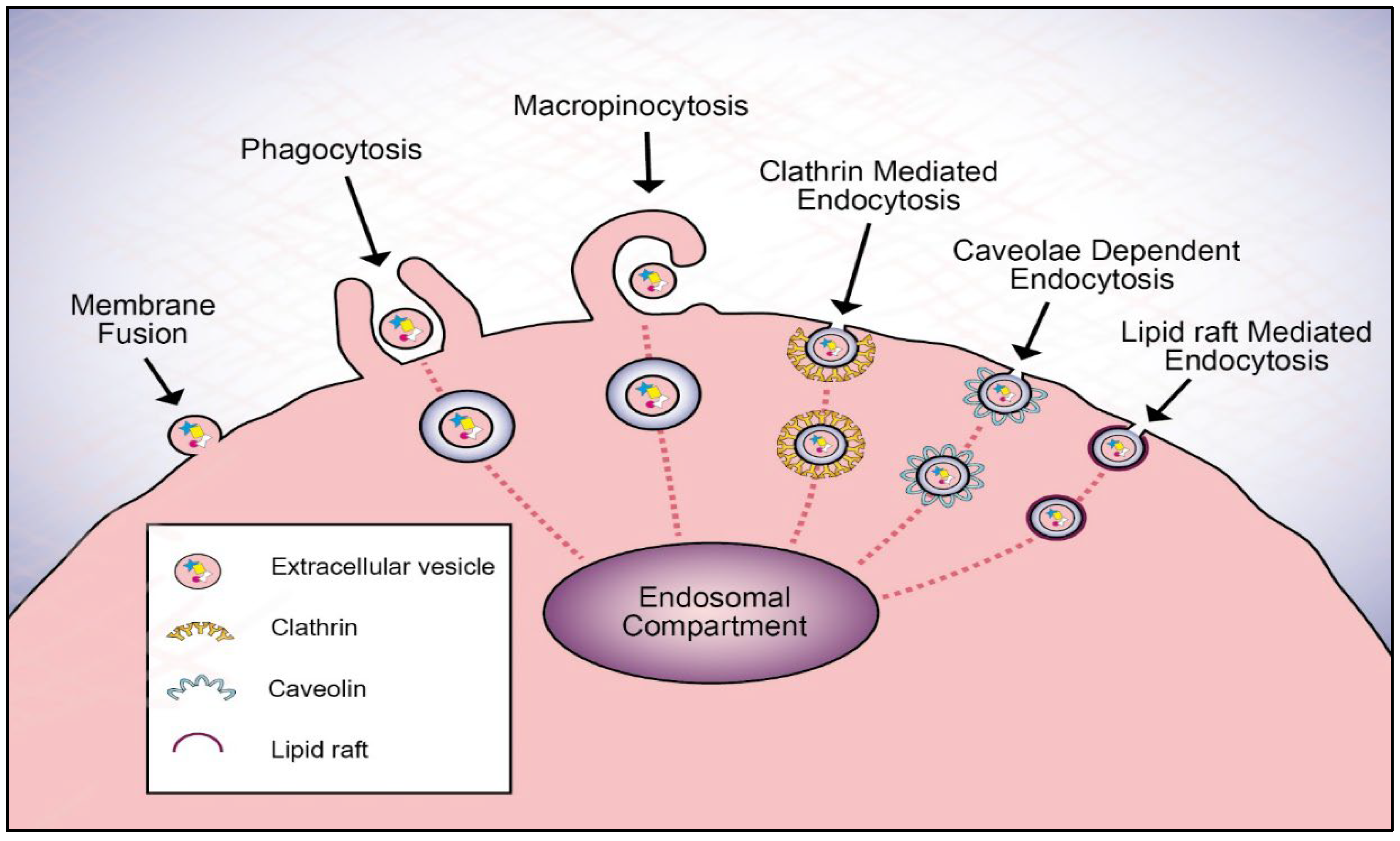The image is a detailed educational diagram with a horizontal rectangular layout, featuring a black border and a faint blue background design. At the lower left corner, there's a white square with a black border that acts as a legend, detailing terms such as "extracellular vesicle," "clathrin," "caveolin," and "lipid raft," each accompanied by an icon. At the center bottom of the diagram is a deep purple oval labeled "endosomal compartment," surrounded by a larger pink semicircle. Red hash marks connect this compartment to multiple round, pink-centered nodules, each pointing to labels such as "lipid raft-mediated endocytosis," "clathrin-mediated endocytosis," "caveolin-dependent endocytosis," "macropinocytosis," and "membrane fusion." The diagram visually represents various cellular processes in a highly medical context.